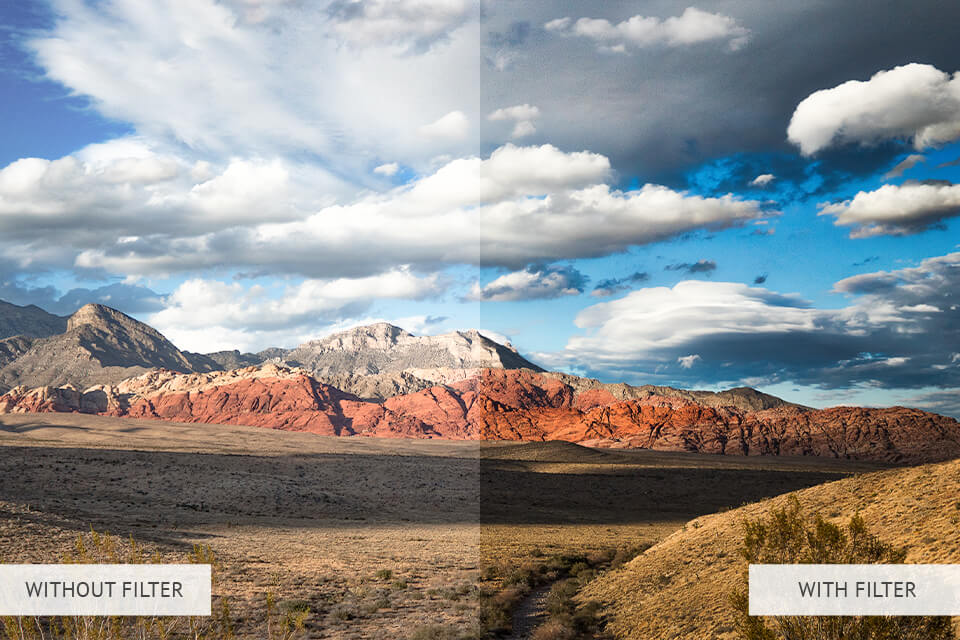This photograph captures a dry, desert-like mountain range, possibly from a region such as Utah or Arizona. The image is distinctly split down the center to compare the effect of a filter. On the left side labeled "without filter," the scenery appears duller but still bright, with puffy white clouds scattered across a blue sky. The desert terrain consists of brown debris and dried brush, reflecting its arid nature. In contrast, the right side labeled "with filter" is notably more vibrant and clear. The clouds appear darker and stormier, enhancing the dramatic effect. The mountains on this side boast richer colors, with visible green foliage in the foreground, offering a striking contrast to the barren landscape of the unfiltered side. The juxtaposition highlights the sharpness and vividness brought out by the filter, creating a more dynamic and colorful view of the same natural setting.